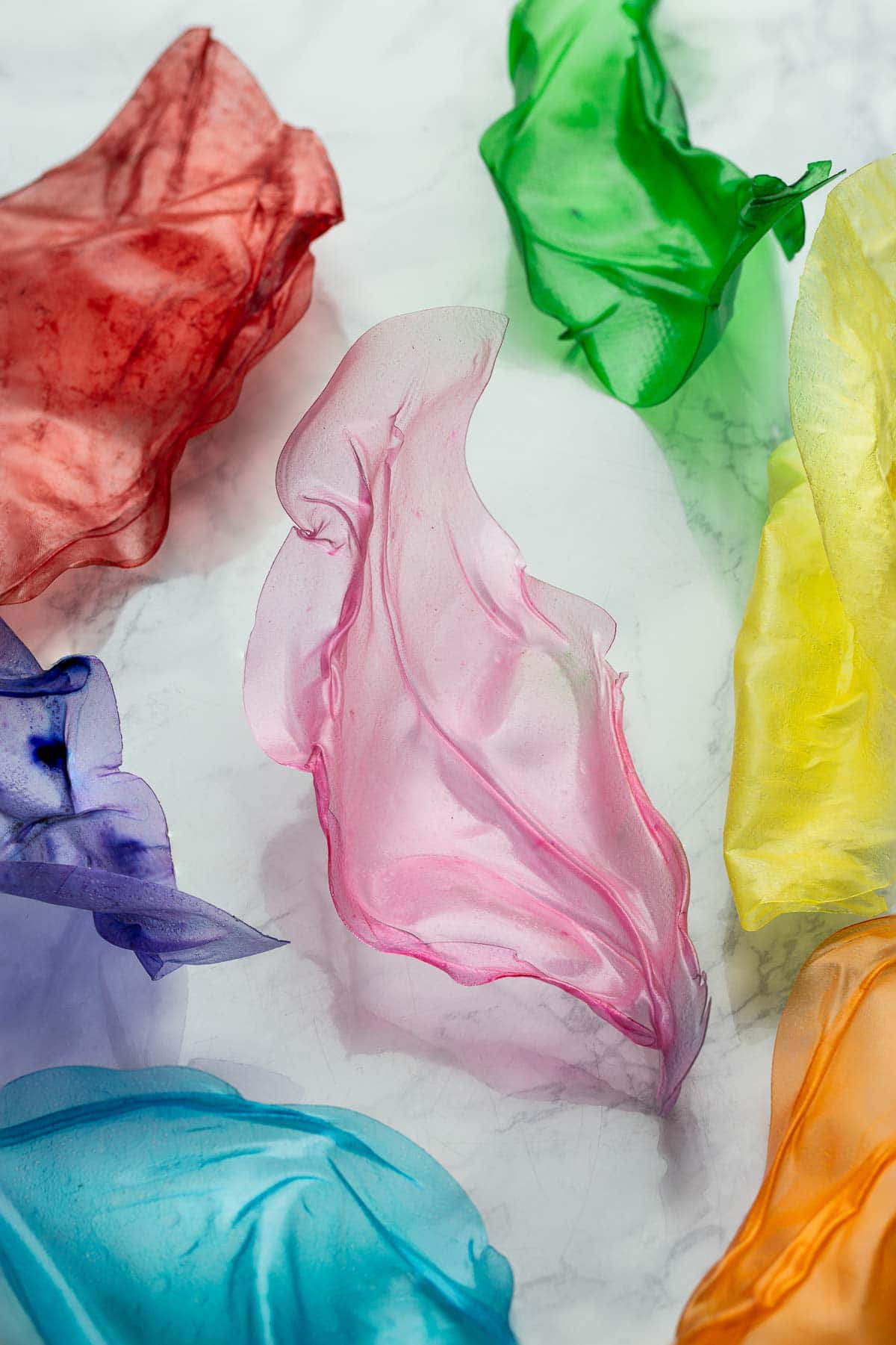This image showcases an intricate artwork of colored blown glass, meticulously arranged on a white granite countertop speckled with gray markings. The glass pieces, resembling delicate, crumpled tissue paper or handkerchiefs, exude a semi-transparent, lucite-like quality that gives an impression of melted leaves or fabric. From top to bottom, the arrangement features a deep red piece on the upper left, a dark green one on the upper right, and a pale pink piece in the center. Flanking the central piece, there is a hint of purple on the left and a light blue piece on the lower left. The bottom is adorned with an orange piece on the right and a vivid yellow piece. The glass, though firm, emanates the texture and appearance of soft, crumpled material, creating an illusion that blurs the line between glass and fabric.